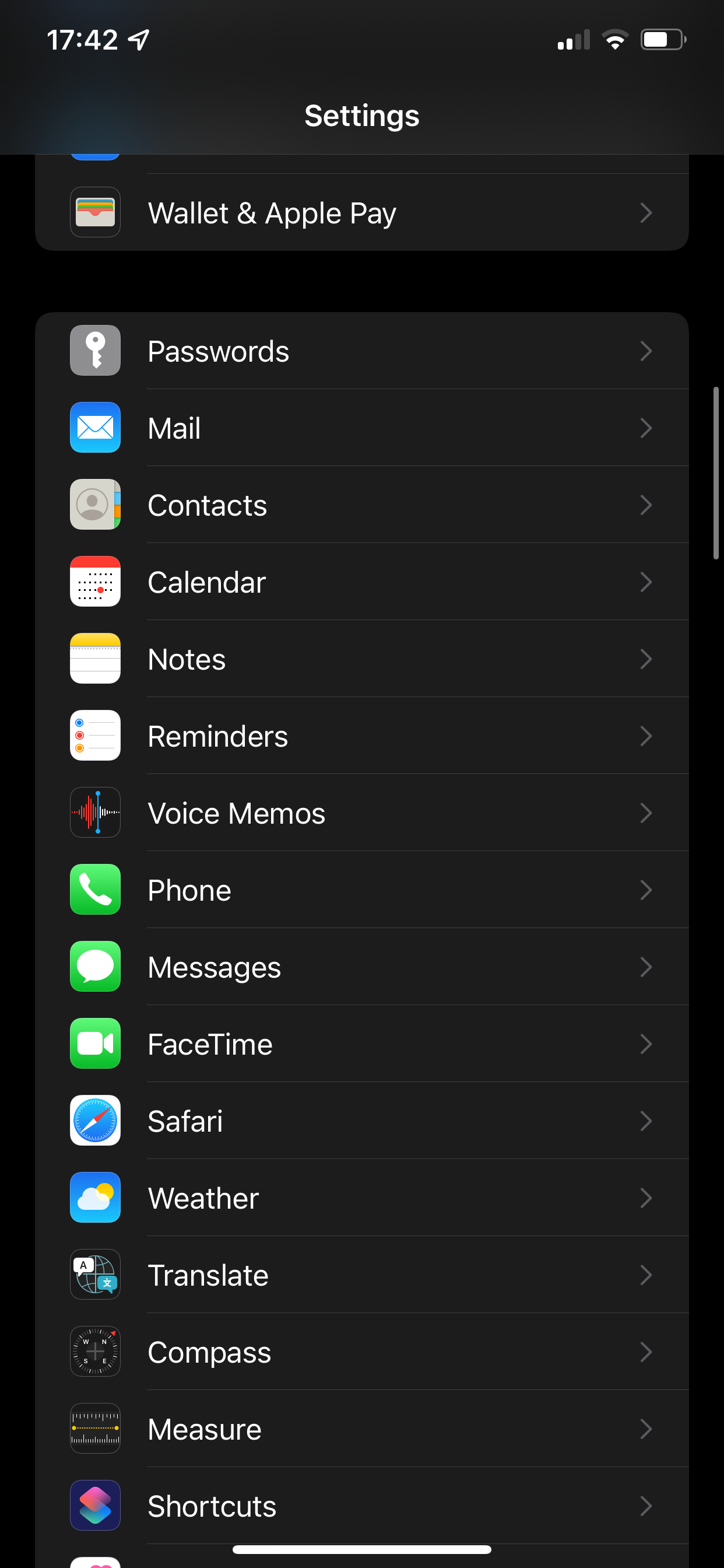This is a detailed screenshot of an iPhone's "Settings" menu, depicted on a black background. The time displayed at the top is 17:42, accompanied by standard icons: an internet connection indicator, a signal strength icon, and a battery charge icon at full capacity. Below the header "Settings," the visible portion of the screen shows the last item in its previous section labeled "Wallet & Apple Pay." Beneath this section, a new section unfolds, predominantly occupying the remainder of the screen.

The new section includes a list of various options, each represented by descriptive icons on the left and right-facing carets on the right. The options are:

1. **Passwords** - No icon detail provided.
2. **Mail** - No icon detail provided.
3. **Contacts** - No icon detail provided.
4. **Calendar** - Icon shows a calendar page highlighting the current month.
5. **Notes** - No icon detail provided.
6. **Reminders** - No icon detail provided.
7. **Voice Memos** - No icon detail provided, correction to "voicemails."
8. **Phone** - No icon detail provided.
9. **Messages** - No icon detail provided.
10. **FaceTime** - Icon represents a video camera silhouette.
11. **Safari** - No icon detail provided.
12. **Weather** - No icon detail provided.
13. **Translate** - No icon detail provided.
14. **Compass** - No icon detail provided.
15. **Measure** - No icon detail provided.
16. **Shortcuts** - No icon detail provided.

This list continues off-screen, with only a partial view provided. Each entry on the list features a rightward-pointing caret, indicating that tapping any item will open a detailed settings submenu for that particular option.